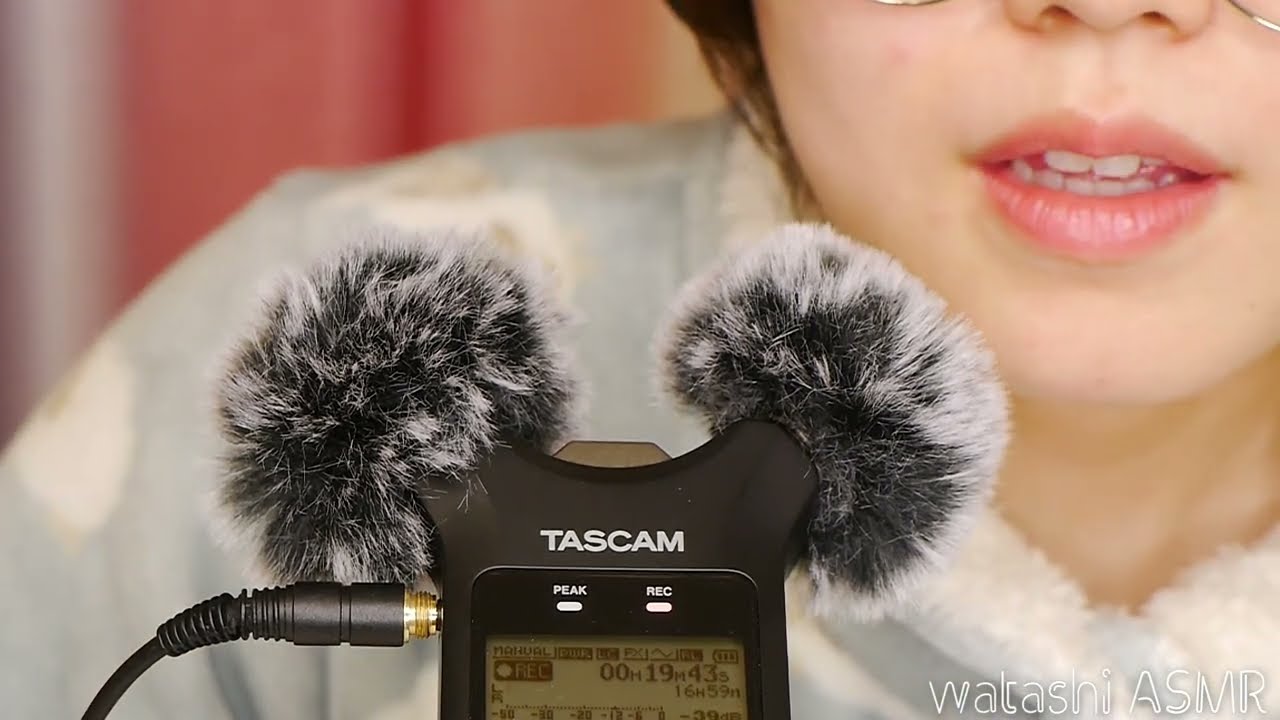The photograph prominently features a TASCAM audio recording system situated in the foreground with a detailed view of its screen displaying "Recording Manual 00H19M43S." The device, identified by the white text labels "PEAK" and "REC," has two fuzzy wind guards on its extensions, resembling ears. A cord is connected to the bottom left of the recorder. In the background, slightly out of focus, is a woman with a light complexion, dark hair, and wire-rimmed glasses. Her face is partially visible, showing her nose, mouth, and slightly open lips as if about to speak, with her upper and lower teeth and tongue slightly visible. She is wearing a white fleece sweater that covers her neck. The background appears blurry with shades of pink and white. In the lower right corner of the image, the text "Walrashi ASMR" is clearly visible, possibly identifying the subject or the content creator.